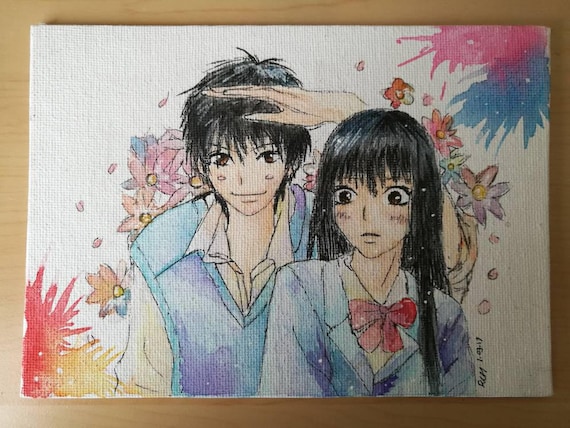The detailed painting portrays two anime-style Japanese characters against a white canvas, seemingly created with either acrylics or watercolor. The central figures, a young Asian male on the left and a female on the right, dominate about 60% of the image. The male character has black, spiky hair partially covering his eyes and wears a blue-purple sweater vest over a cream-colored, open-collar button-down shirt. He displays a half smile and raises a hand to shield his eyes from light. The female character, positioned on his right, features long dark hair with fringy bangs, large, raised eyes with a slight frown, and a worried expression. She dons a blue blazer with a red bow tie at her neck. Surrounding them are various light color washes and star-shaped splashes of purples, blues, and yellows. Notably, a burst of pink and blue accents the top right corner, while orange and red hues splash along the bottom left, complemented by purple and red flowers adjacent to the female character. The painting is set on a gold-colored wooden background, emphasizing its manga-style anime art form.